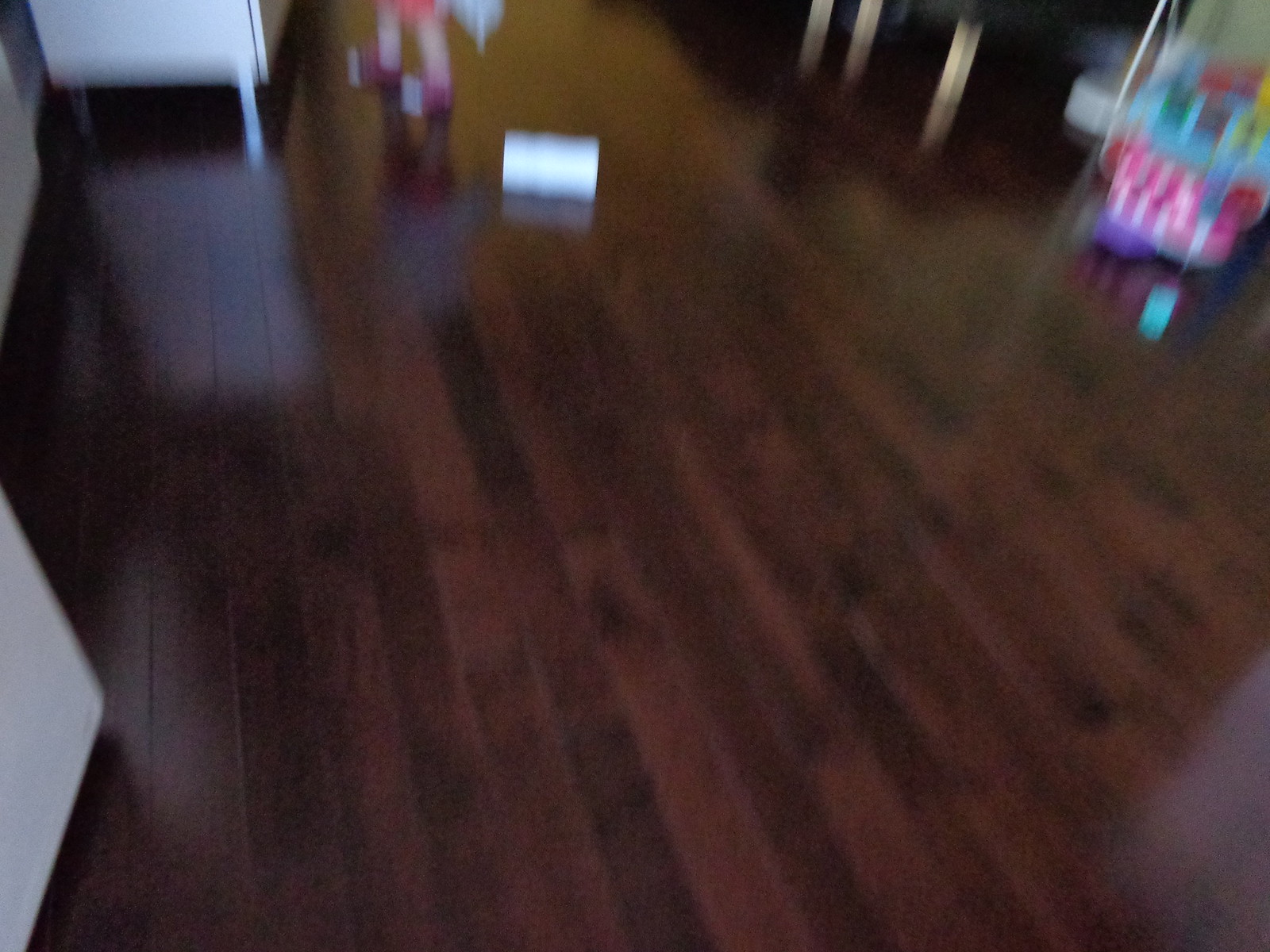This color photograph is noticeably out of focus, likely taken with the camera in motion. The image predominantly captures an indoor scene with a dark-stained wooden floor stretching across the frame. On the left side of the photo, partially visible and blurry, are what appear to be white cabinets, suggesting the setting might be a kitchen or similar area. Despite the lack of clarity, the composition hints at a cozy interior space characterized by its rich flooring and light cabinetry.